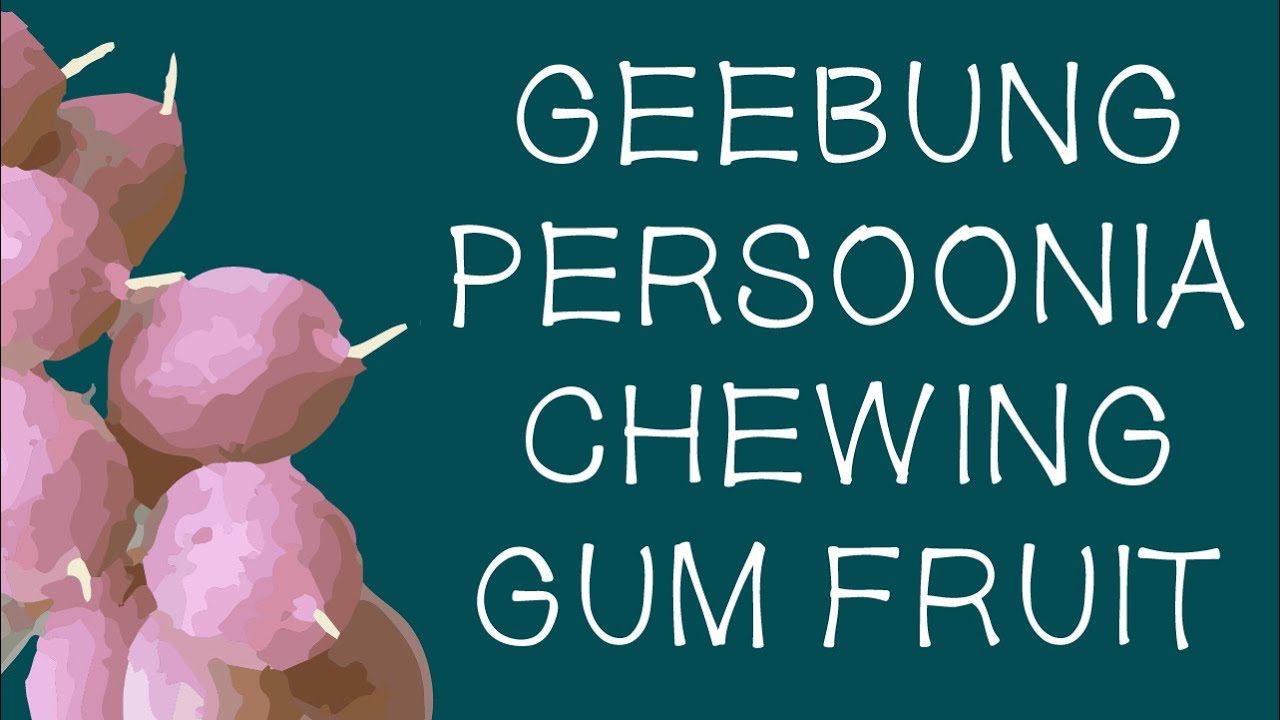The image features a long, horizontal, dark teal background with a detailed arrangement of text and imagery. On the left-hand side, there are illustrations of fruits resembling purple grapes with white accents and short white stems. These fruits are spherical to oval in shape, and while they look similar to lychees with their pinkish hue, they lack the characteristic spiky exterior. On the right-hand side of the image, there are four lines of text in all-white capital letters. At the top, it reads "GEEBUNG," followed by "PERSUNIA," "CHEWING," and "GUM FRUIT." Notably, this detailed depiction of various colors and textures combines to create an intriguing visual representation of an unknown fruit described as "Geebung Persunia Chewing Gum Fruit."